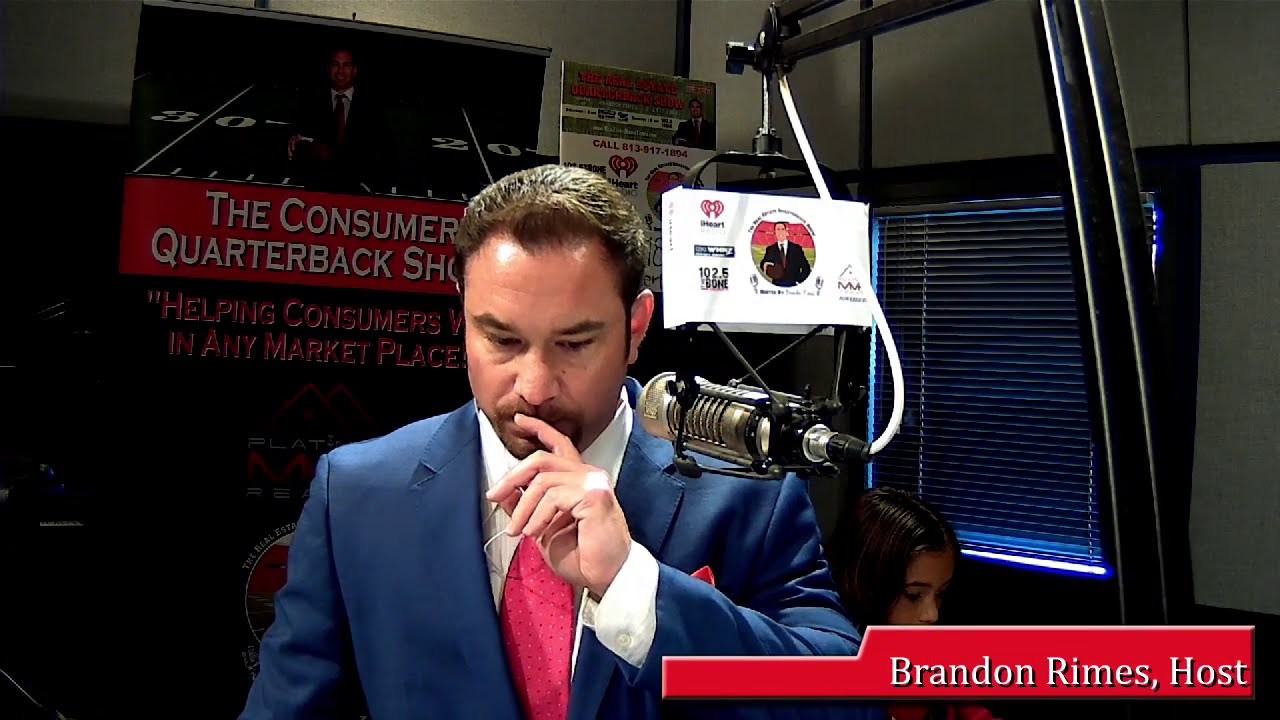In this image, a man identified as Brandon Rimes, the host of a show, is captured midway through what appears to be a podcast or radio interview. He stands in front of a silver microphone labeled with "102.5 The Bone" and "sponsored by iHeart." Brandon is clad in a sharp blue suit, complemented by a white dress shirt and a red patterned tie, accentuating his professional attire. His short brown hair and a brown goatee frame his thoughtful expression as he rests his left forefinger against his lips. 

The setting suggests he could be discussing topics related to consumer advice, as indicated by a partially visible poster behind him emblazoned with "The Consumer Quarterback Show" and the phrase "helping consumers in any marketplace." The room features white walls with a black border, and a window with closed blinds to the side.

In the background, a woman with long, straight brown hair is partially visible, suggesting she is a guest or co-host. She seems to be seated, further contributing to the dynamic atmosphere of this apparent studio setting.